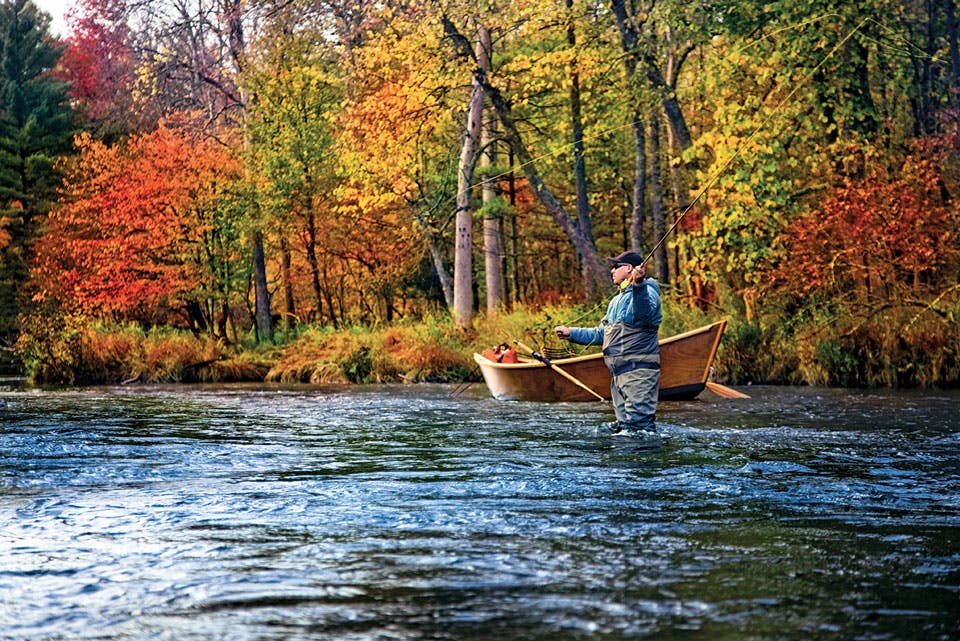In this vibrant fall afternoon scene, a man stands knee-deep in a calm, gently flowing river, fly-fishing with focused precision. He is attired in green waders and a blue hooded jacket with a black lower half, complemented by a baseball cap, sunglasses, and earphones. His left hand skillfully manages the reel as he casts his line. The serene, natural beauty around him is illuminated by bright daylight, showcasing a tapestry of autumn foliage. Trees on the riverbank display a stunning array of colors, transitioning from deep green to vivid yellow, orange, and red. Behind him is a wooden canoe with distinct natural staining and a black base, anchored peacefully with paddles in the water. Inside the canoe, a red bag and an orange life preserver can be spotted. This picturesque setting, with its mix of vibrant foliage and serene water, captures the essence of a tranquil autumn day perfect for fly fishing.